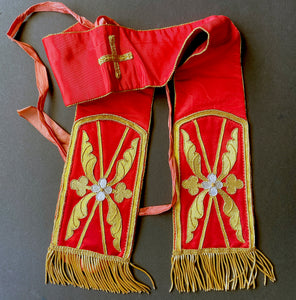This image depicts a vibrant, bright red scarf-like garment, likely used as part of a priest's attire for religious ceremonies, presumably within the Catholic tradition. The garment is designed to be draped over the shoulders and features elaborate embroidery. Each end of the scarf is adorned with identical intricate designs: white berries with golden leaves extending outward, framed by a thin golden border. The garment's ends are finished with lush golden tassels. Central to the piece is a prominent golden cross embroidered at the midpoint, aligning with where the garment would rest at the neck when worn. The scarf is displayed on a gray table, highlighting its rich colors and detailed craftsmanship.